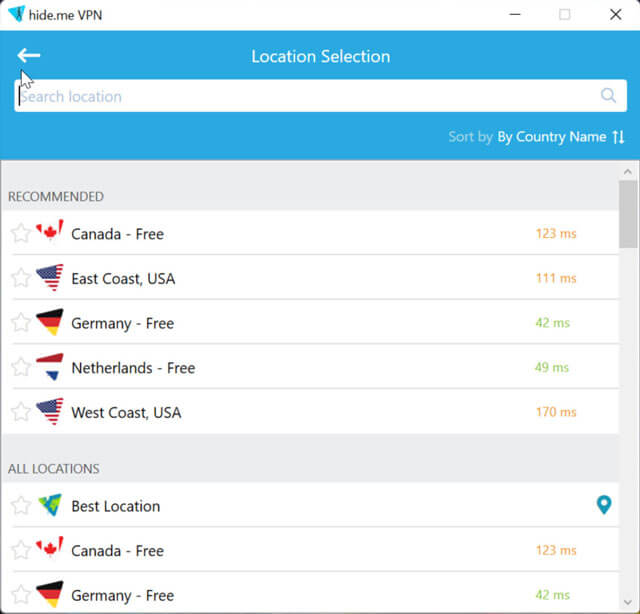This is a detailed description of a VPN site map displayed via a screenshot on a mobile phone. 

At the top left corner of the interface, there is a teal-colored triangle containing a small black silhouette of a stick figure. Next to this, the text "Hide.meVPN" is displayed prominently. Further to the right, there are standard minimize, maximize, and close buttons.

Below this top section, a light sky blue bar appears with the text "Location Selection" in white, accompanied by a back arrow to the left side of the text. Below this bar is a search bar labeled "Search Location," marked with a magnifying glass icon.

Following the search bar, the text "Sort by Country, Name" is featured, along with up and down arrows for sorting options.

The next section is titled "Recommended" and lists various VPN server locations with details:
- "Canada Free 123 MS" with a small triangle (resembling a Dorito) displaying the Canadian flag, and unfilled stars to the left. The "123 MS" is shown in orange, indicating latency over 100 ms.
- "East Coast USA 111 MS" with the USA flag and unfilled stars, the "111 MS" also in orange.
- "Germany Free 42 MS" with the German flag and unfilled stars, the "42 MS" in green indicating latency under 100 ms.
- "Netherlands Free 49 MS" with the Dutch flag and unfilled stars, the "49 MS" in green.
- "West Coast USA 170 MS" with the USA flag and unfilled stars, the "170 MS" in orange.

Additionally, under a section labeled "Best Location" marked with a location pin icon:
- The same details for "Canada Free 123 MS" and "Germany Free 42 MS" are reiterated.

Each listed country appears in black text, and latency (MS) is color-coded: green for under 100 ms and orange for over 100 ms.